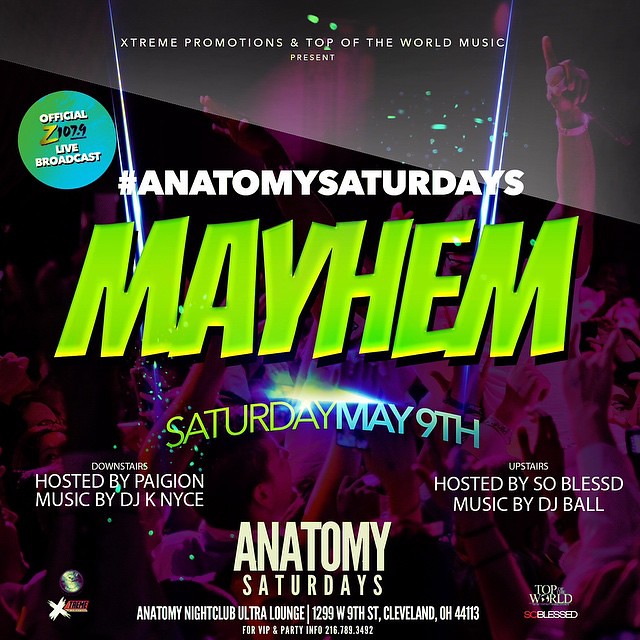Promotional graphic for Anatomy Nightclub's event, "Anatomy Saturdays Mayhem," hosted on Saturday, May 9th at 1299 West 9th Street, Cleveland, Ohio, 44113. The vibrant background features concert-goers with hands raised, basked in a purplish-pink hue. The event promises a dynamic night with the downstairs hosted by Pajeon and music by DJ K Nice, while upstairs is hosted by So Bless with DJ Ball. Highlighted prominently in large green letters is the word "Mayhem." The top of the image notes "Extreme Promotions and Top of the World Music Present," along with a live broadcast by Official Z107.9. For VIP and party details, call 216-789-3492. Logos from Top of the World and Z107.9 are also featured within the design, encapsulating the high-energy and festive atmosphere of the event.